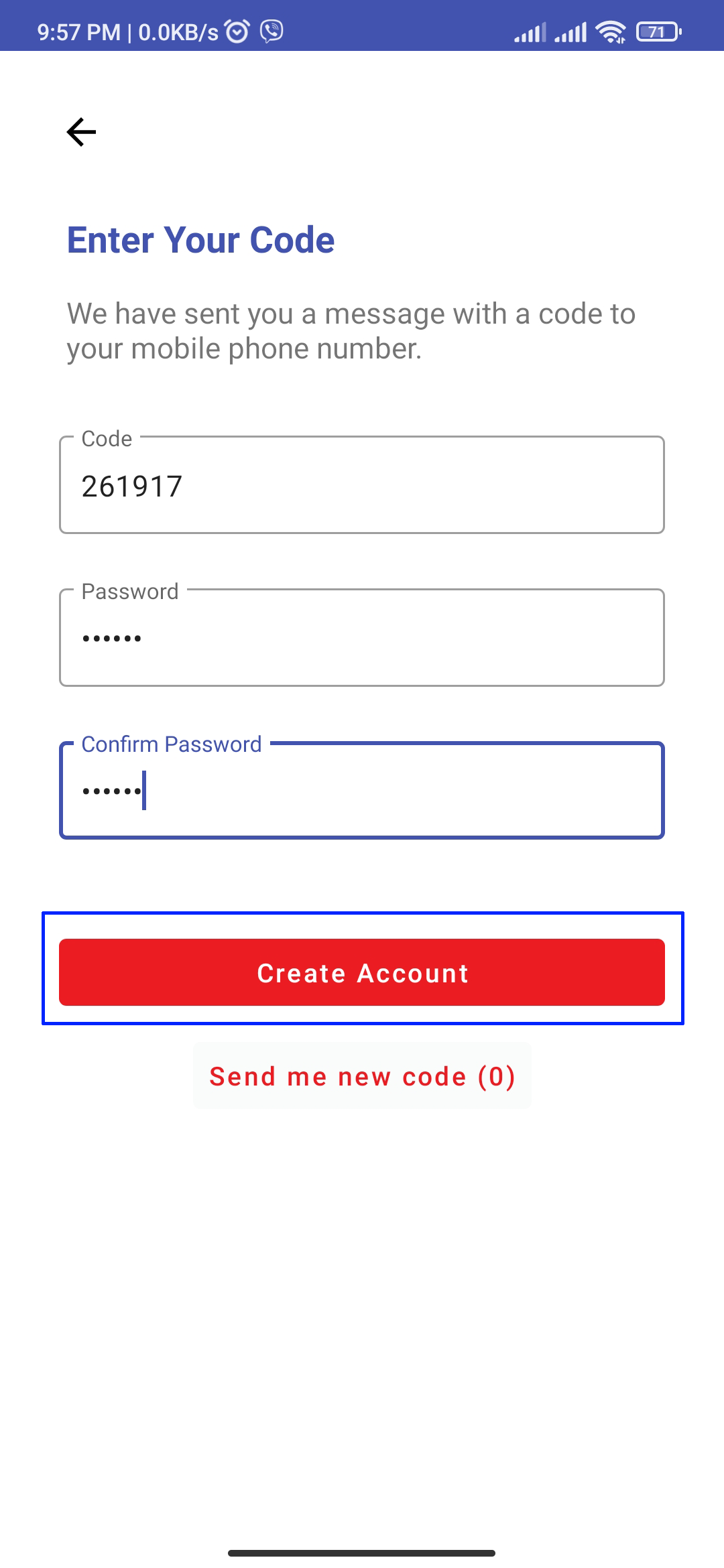A screenshot from a phone displays various device statuses, including two signal bars, active Wi-Fi, and a battery level at 71%. The time is 9:57 PM, and data transfer is at 0.0 kilobytes per second. Notifications show active alarms and a missed call.

The screenshot captures a verification page for creating an account. At the top, there's a back button. Below, the text "Enter your code" is highlighted in blue, followed by gray text stating, "We have sent a message with the code to your mobile phone number." An input field is pre-filled with the code "261917."

Further down, there are fields for entering and confirming a password, both represented by dots for security. At the bottom, a red "Create Account" button with a white text label is outlined in blue. Additionally, there's an option to request a new code in red text that says "Send me a new code (0)." 

The screenshot suggests that the user is in the process of verifying their identity via a code sent to their mobile phone to complete the account creation process.